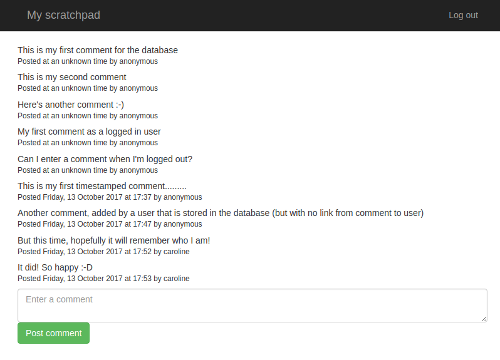The image features a personal diary interface titled "My Scratchpad" prominently displayed at the top center of the screen in a light gray font against a black background. On the far right of the title bar is a faded "Logout" option. The main content area consists of two left-aligned paragraphs, slightly blurred, making the text difficult to read. However, some words are decipherable, indicating it is a user-generated comment on a database, posted by "Anonymous." Below the main content, there is a white comment section box with the placeholder text "Enter Comment" in a faded font. This box includes a small arrow in the bottom right corner, suggesting it can be resized. Beneath this box, there is a green button labeled "Post Comment." The overall layout hints at a user-friendly design aimed at facilitating diary entries and subsequent comments.